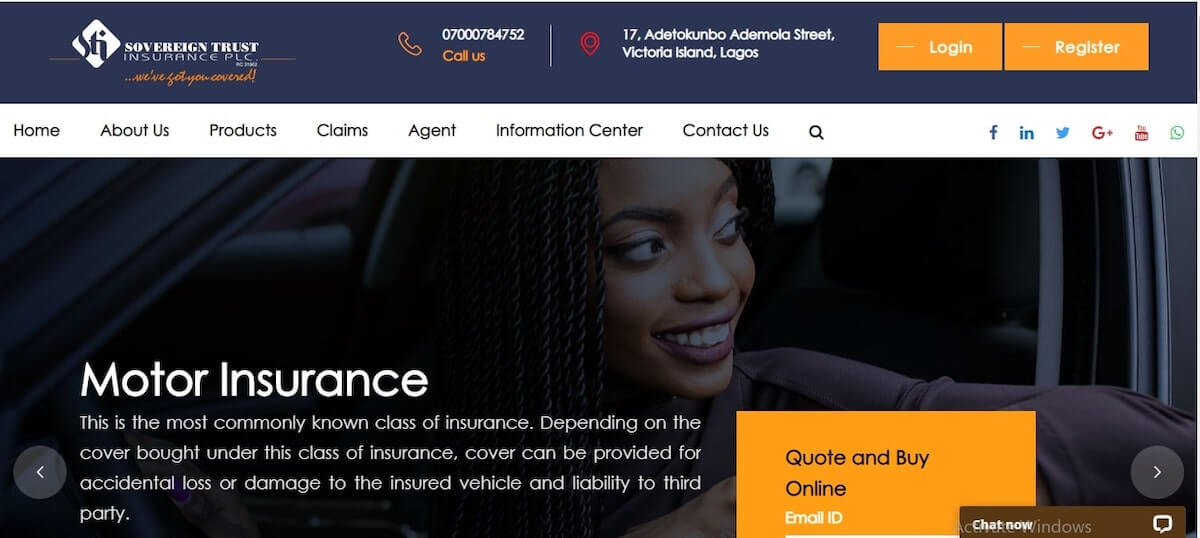Screenshot of Sovereign Trust Insurance PLC Website:

The top section of the screenshot features a dark bluish-black bar containing various company details. On the left side, there's the company logo, a white diamond shape with the letters "STI" in black, set against the same dark background. Adjacent to the logo is the company name, "Sovereign Trust Insurance, PLC," followed by their tagline in orange cursive text: "We've got you covered."

Next to this, there is an orange phone icon with the company's contact number beside it, labeled "Call Us" in orange. The address is also displayed nearby, marked with a red Google Maps pin icon. Towards the right side of this bar, two orange boxes offer options to "Login" and "Register."

Beneath this, a white navigation bar provides links to different sections of the website, with social media icons aligned to the right.

The main portion of the image focuses on a promotional banner. The background shows a close-up of a black woman with dark hair, wearing a purple shirt, seated in a car. Overlaid on this image is large white text that says "Motor Insurance." Below this, a detailed description reads: "This is the most commonly known class of insurance. Depending on the cover, this class of insurance can provide for accidental loss or damage to the insured vehicle and liability to third parties."

An orange box below this text invites users to "Quote and Buy Online." The image cuts off before the start of the user information input section, which begins with a field labeled "Email ID." Navigation arrows in grey circles are present on either side of the promotional banner, indicating additional options that can be viewed by scrolling.